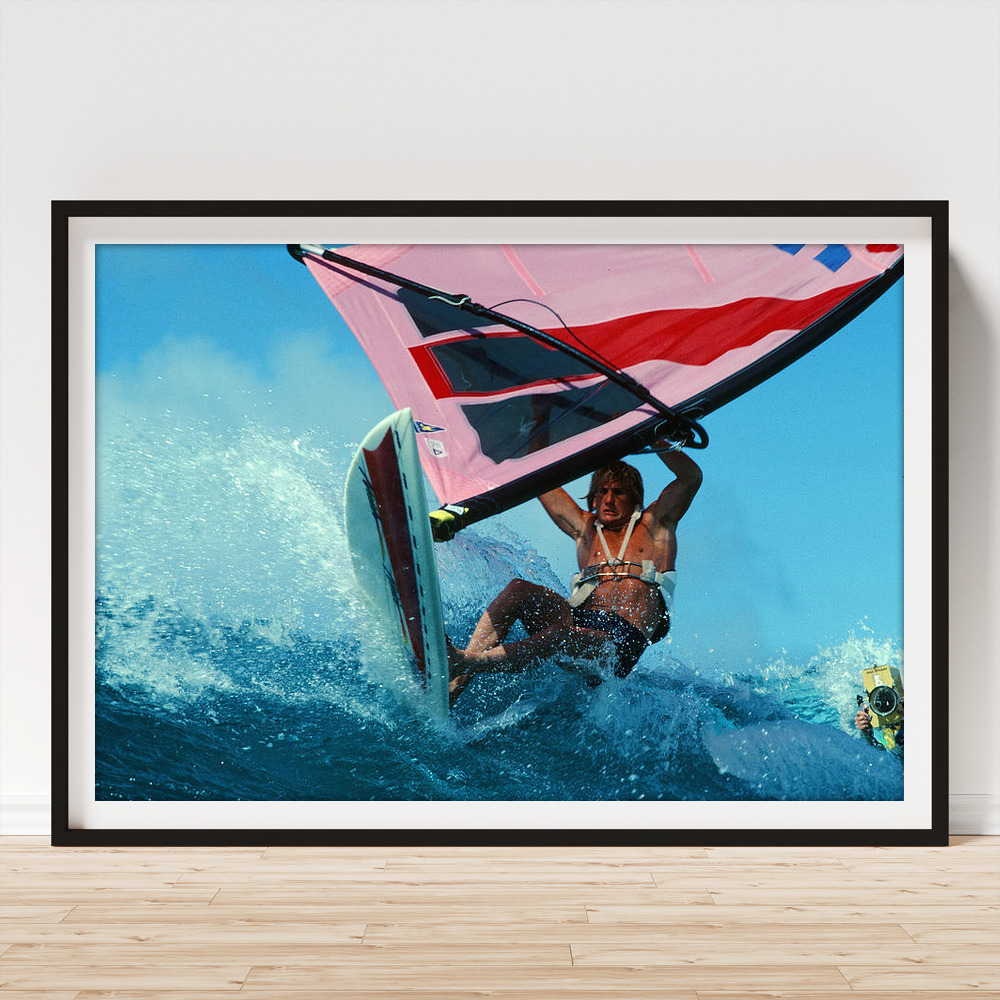In this vivid photograph, a man is captured engaging in a thrilling watersport on the ocean. He is skillfully maneuvering on a white surfboard marked by a distinctive brown stripe. The front of the surfboard is arched upward out of the water, creating a dramatic splash. He is gripping a hydroplaning windsurfing apparatus, demonstrating intense physical exertion as evidenced by the strain on his face. He wears a secure life jacket, ensuring his safety during the high-energy activity. His legs appear shadowed, adding to the dynamic lighting of the scene. The bright blue sky serves as the perfect backdrop to this moment of concentrated action. In the distance, another individual can be seen with a camera, meticulously capturing the exhilarating experience either through video or photographs.